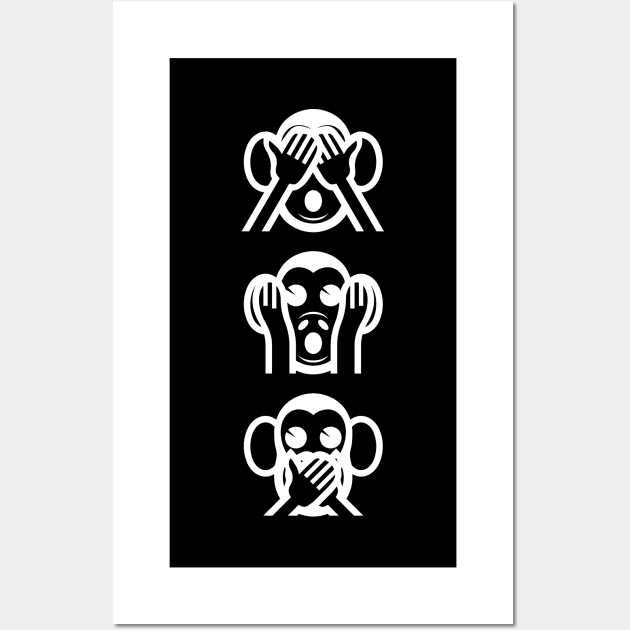The image features a square photograph taken indoors, measuring approximately 4-5 inches on each side. It is mounted against a gray wall, bordered by white borders about half an inch wide. Within this frame, there is a black vertical rectangle, measuring roughly 2-1/2 inches high and 1-1/2 inches wide. The black rectangle contains minimalist white outlines of three monkey heads arranged vertically. The top monkey covers its eyes, the middle one covers its ears with wide-open eyes and an 'O' shaped mouth, and the bottom monkey covers its mouth. These positions respectively represent the "See No Evil, Hear No Evil, Speak No Evil" motif. The artwork is presented in a clean and simple style, emphasizing the iconic gestures through a high contrast between the black background and white outlines.